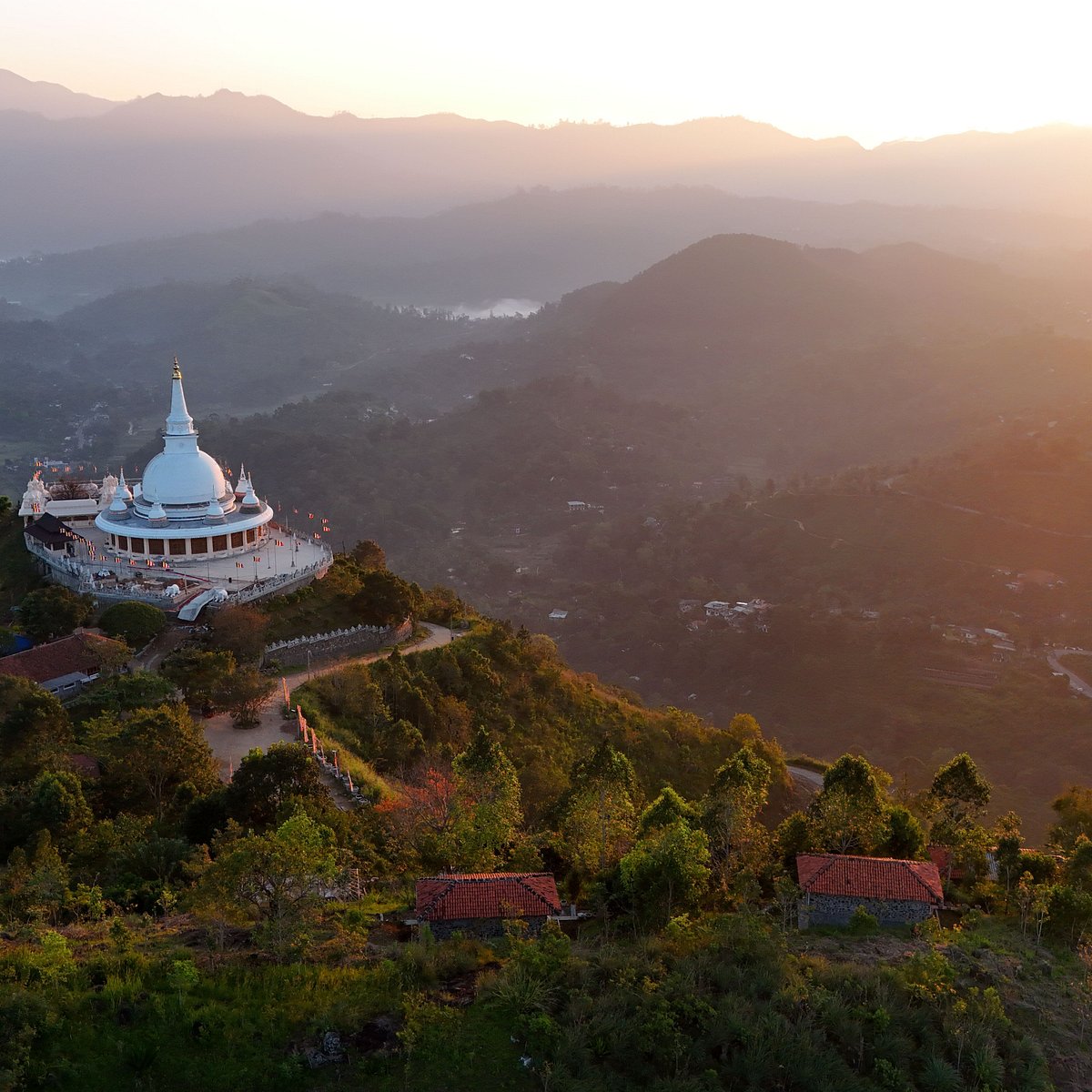The color photograph captures an overhead view of an Asian temple complex situated on a hilly mountain range. The focal point is a white domed building with a prominent spire capped in gold, surrounded by smaller spires that replicate this design. The temple is adorned with red and white flags that flutter from numerous poles encircling the structure. Flanking the entrance are statues of animals, likely tigers, adding to the grandeur. A winding paved road and a walk-up trail lead to the temple, which is nestled among lush green trees and bushes. In the bottom left, the roofs of two small buildings with red clay tiles are visible. The background features a vast mountain range shrouded in a foggy atmosphere, while a bright yellow sky illuminates the top of the scene, with sunlight piercing through the upper right corner.